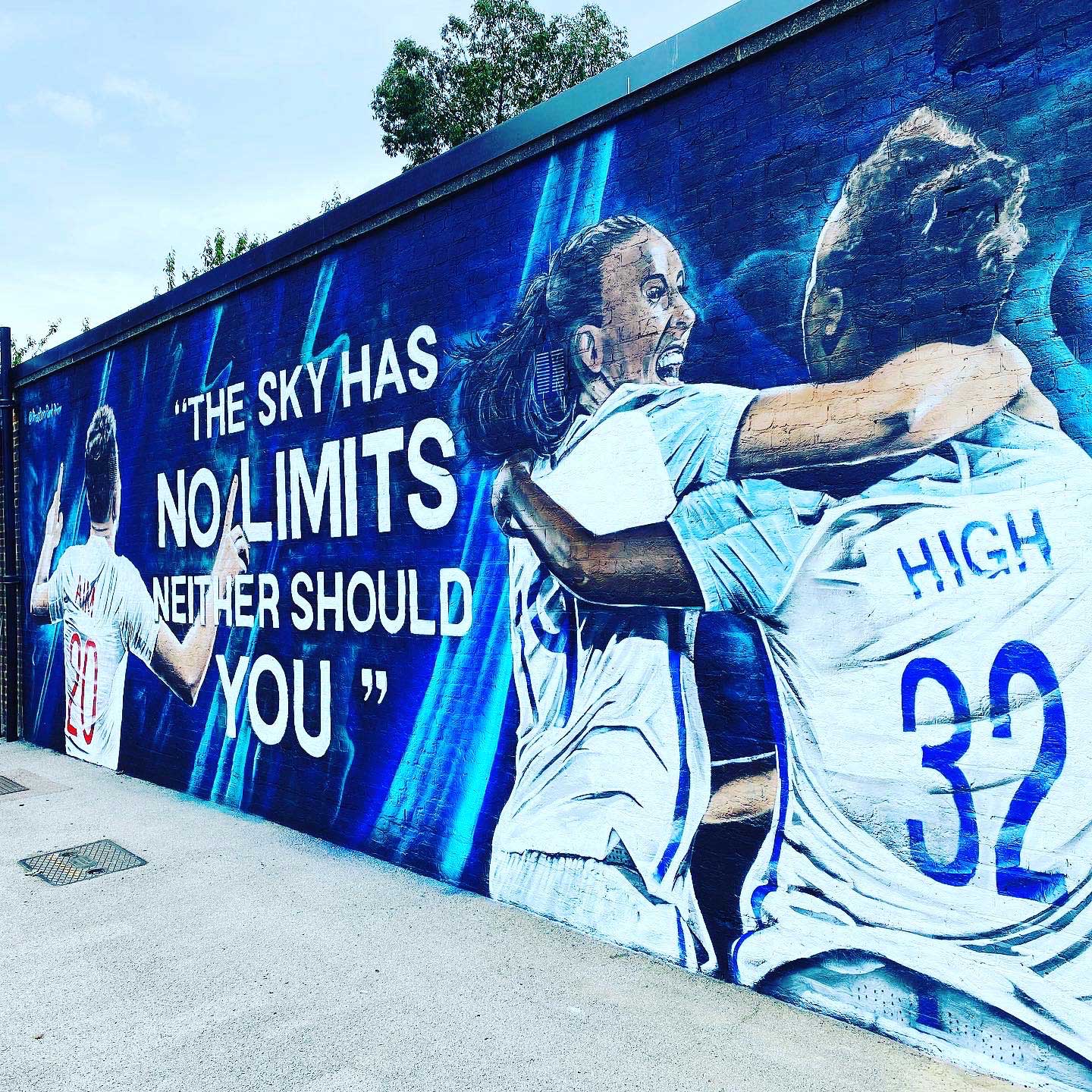This photograph captures a vibrant mural painted on a brick wall with a gray concrete floor at its base. The mural features a bold blue background with intricate lines, highlighted in white. The centerpiece of the artwork is a motivational quote in white text with a black outline, stating, "The sky has no limits, neither should you." To the left of the quote, a male figure with the number 20 on his jersey stands with his back to the viewer, arms raised and one finger pointing upwards in celebration.

On the right, two athletes, a black woman and a white woman, are depicted embracing joyfully. Both are clad in white jerseys with blue stripes, and the black woman's jersey reads "HI" with the number 32, while the white woman's jersey displays the number 19. The detailed expressions show them smiling broadly. This mural, with its diverse characters and powerful message, exudes a sense of unity and limitless potential, likely situated near a school or a sports field, given its inspirational and athletic themes.